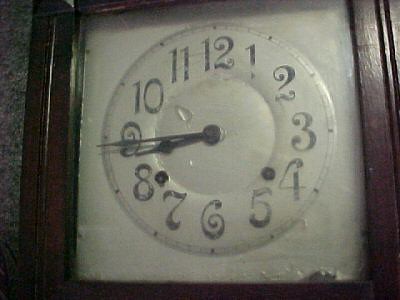This photograph showcases an old-fashioned, square-shaped wall clock bordered by dark brown painted wood. The clock features a white, slightly chipped background, particularly noticeable along the bottom edge. Within the square frame, the clock face itself is round, with black numerals written in a standard font. The hands of the clock—black for both the hour and minute—indicate the time as approximately 8:44, or a quarter to nine. A few drops of water are visible on the clock face, along with some scratch marks on its surface. The clock is set against a speckled backdrop resembling white, gray, and black granite or a wall with dotted patterns.